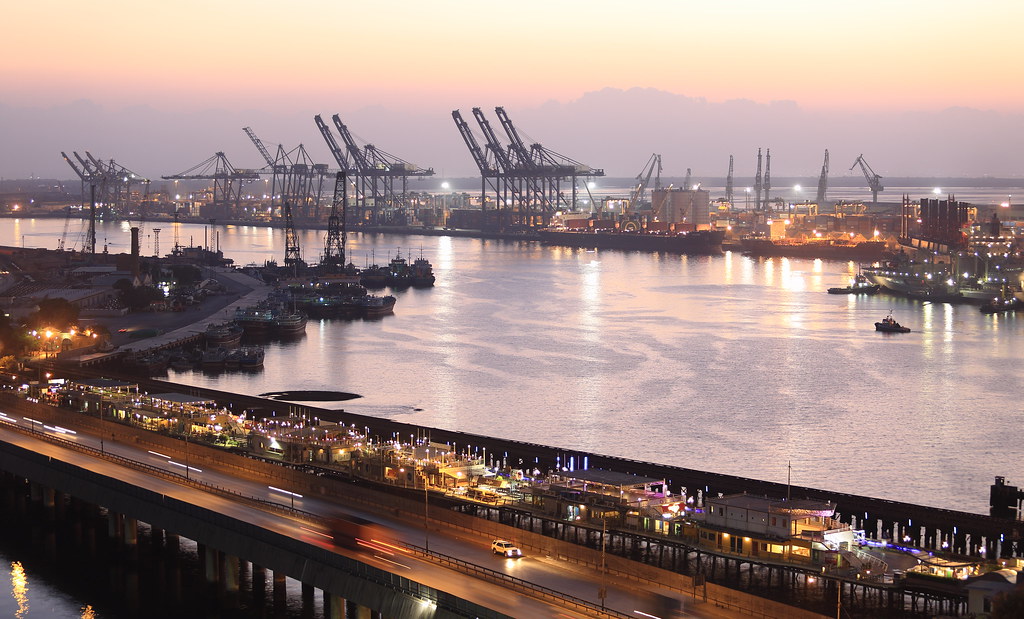This photograph, taken during the twilight hours of either evening or early morning, captures the bustling yet tranquil ambiance of a large city center adjacent to a major harbor. A prominent feature of the cityscape is a substantial bridge with dark gray or black roads that resemble a two-lane highway. Sparsely trafficked, the bridge is supported by numerous concrete pillars that emerge from the water below. On the left, the water appears in various shades of gray, interspersed with white lights reflecting off the buildings, creating a captivating interplay of light and shadow.

On the right side of the bridge, a dense array of illuminated buildings flanks the highway, adding a vibrant touch to the scene. In the distance, a large factory also stands aglow, contributing to the city's industrial charm. The harbor, bustling with maritime activity, houses several ships on the right side, highlighted by one particularly large vessel that stands out, its lights twinkling in the twilight. 

On the left side of the harbor, a conglomeration of smaller ships, predominantly tugboats, are nestled close to three prominent loading cranes. Further into the background, rows of colossal loading cranes dominate the horizon, with some grouped in sets of three, hinting at the extensive freight operations supported by the harbor. These cranes are silhouetted against a dramatic sky that transitions from gray to a fiery orange-red before fading into dark gray and black hues.

The water on the right side of the image is a lighter gray, marked by ripples of darker gray and adorned with a multitude of reflected lights. The contrast between the industrial elements and the serene water, coupled with the dramatic sky, encapsulates the dynamic yet serene essence of this metropolitan harbor scene.